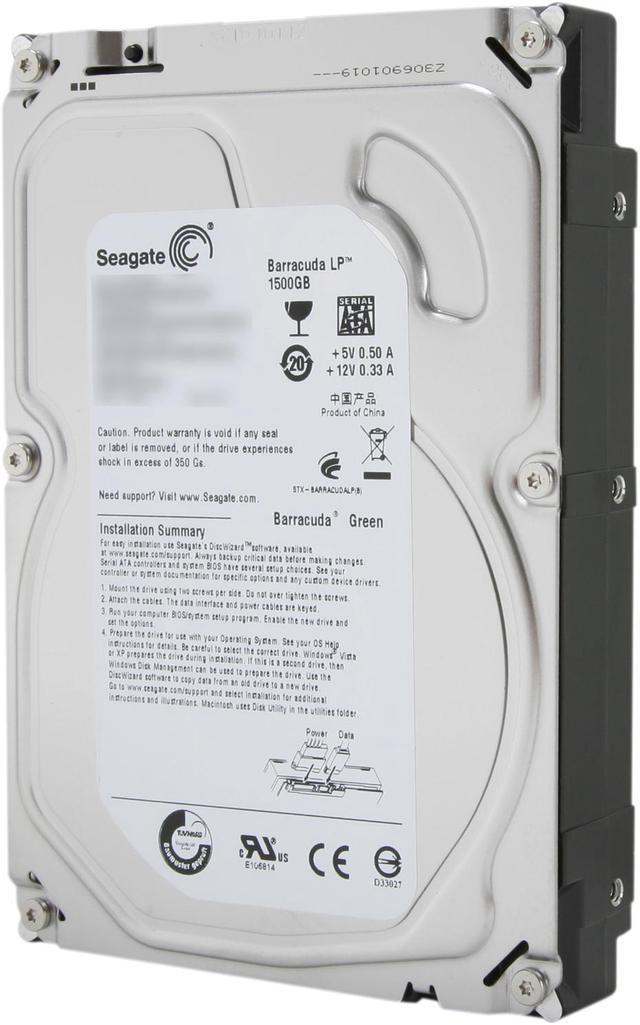The image depicts a large, rectangular electronic device, most likely a Seagate Barracuda LP hard drive with a capacity of 1,500 gigabytes. This device, commonly utilized in computers for storage, features a gray-colored exterior and stands vertically with a bottom view visible. The faceplate is metal with a slightly circular bottom part and a rectangular top part, and the sides are dark gray or black.

Key details include:
- The brand name "Seagate," accompanied by a swirling line logo.
- A large label indicating "Barracuda Green," the product capacity of 1,500 GB, and power requirements of 5 volts or 12 volts, denoting it as a product made in China.
- Several instructions and an "Installation Summary" in fine print.
- Three input holes and six T-star screws (four at the corners and two on the sides), anchoring the device.
- Smaller identifiable elements such as the letters "C" and "E" in a split, cursive style at the bottom, and a large label reading "C8."
- The exterior features dark gray with silver fasteners and a grayish white-colored base, indicative of its practical, sturdy design necessary for housing internal electronic components.

These elements together confirm its robust design suited for internal use within computing systems, providing substantial storage capacity and reliable performance.